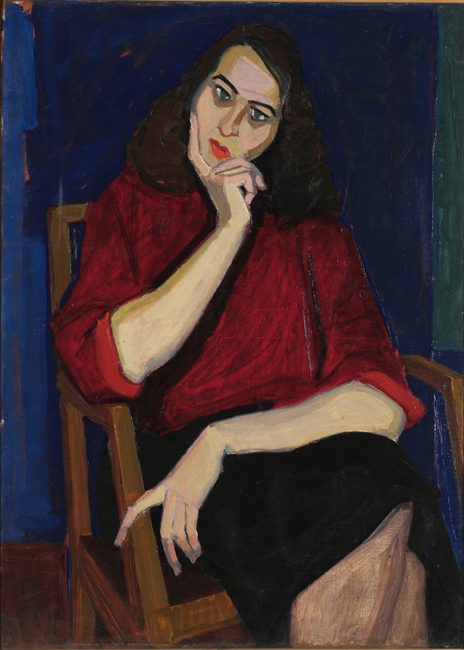This image showcases a woman seated in a simple brown wooden chair against a dark blue background. She wears a dark red shirt with rolled-up sleeves and a black skirt, her legs crossed demurely. Her brown, mid-length hair frames her face, emphasizing her green eyes and red lipstick. Her left hand rests on her lap with one finger pointed, while her right hand supports her chin in a thoughtful posture, with her head slightly tilted to the left. The painting style is simplified and two-dimensional, with smooth, solid colors that clearly define her features, giving her an almost interrogative or stern expression. The floor beneath her is a simple brown, further highlighting the minimalist and focused composition of the artwork.